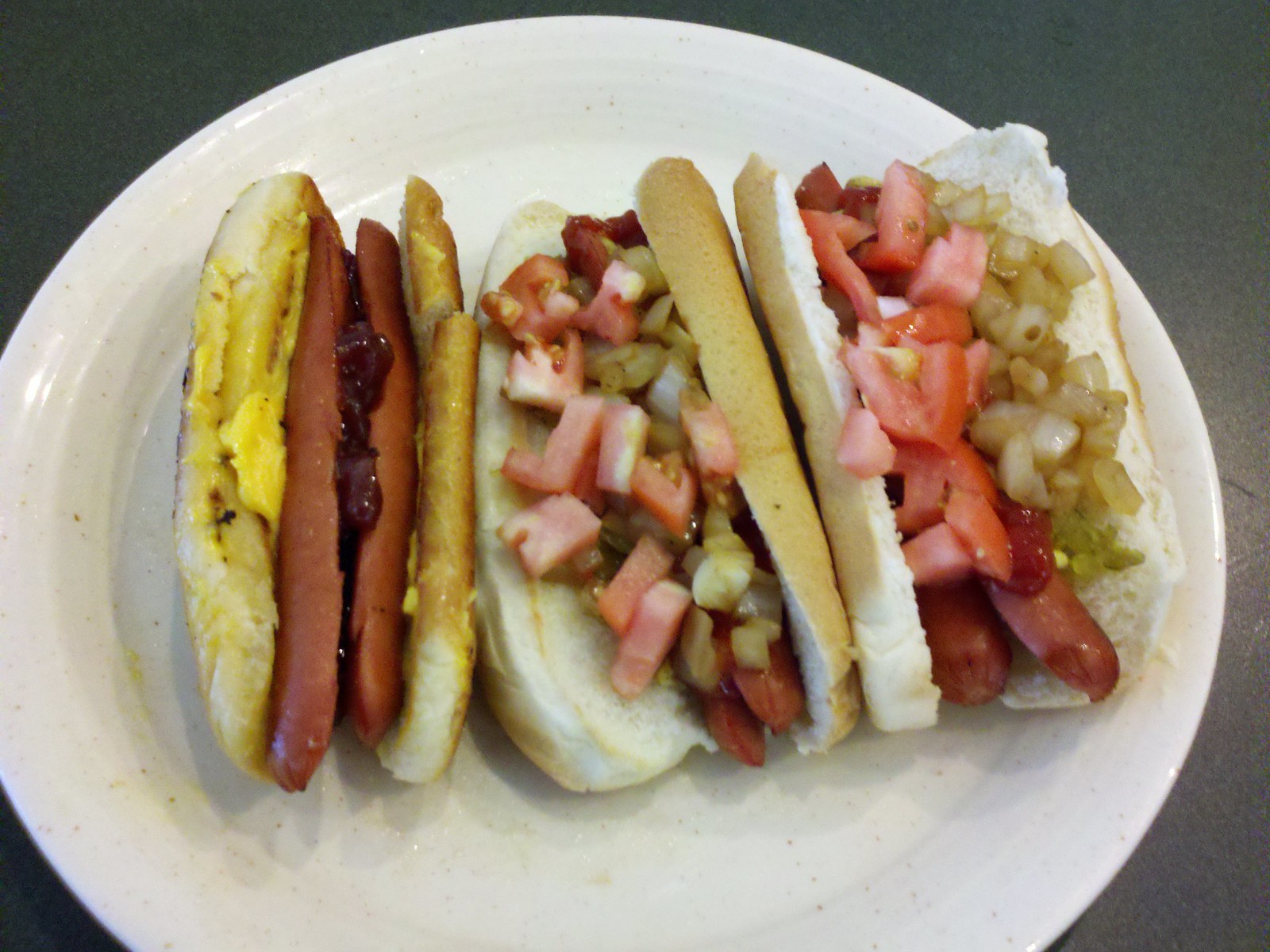In this detailed image, a white, circular plastic plate rests atop a dark gray table. The focus is on a trio of hot dogs, each nestled in a bun. The background is a mix of dark gray, slightly visible at the edges of the image. 

Starting from the left, the first hot dog is sliced in half and dressed with condiments—ketchup in the center, flanked by mustard on either side. The middle hot dog features toppings of chopped tomatoes and green slices, possibly onions or another garnish. Similarly, the hot dog on the right is adorned with tomatoes and a similar lightish yellow-green slice, and appears to contain two hot dogs within the bun. The overall composition centers on the hot dogs, creating a vibrant and appetizing display against the neutral-colored setting.